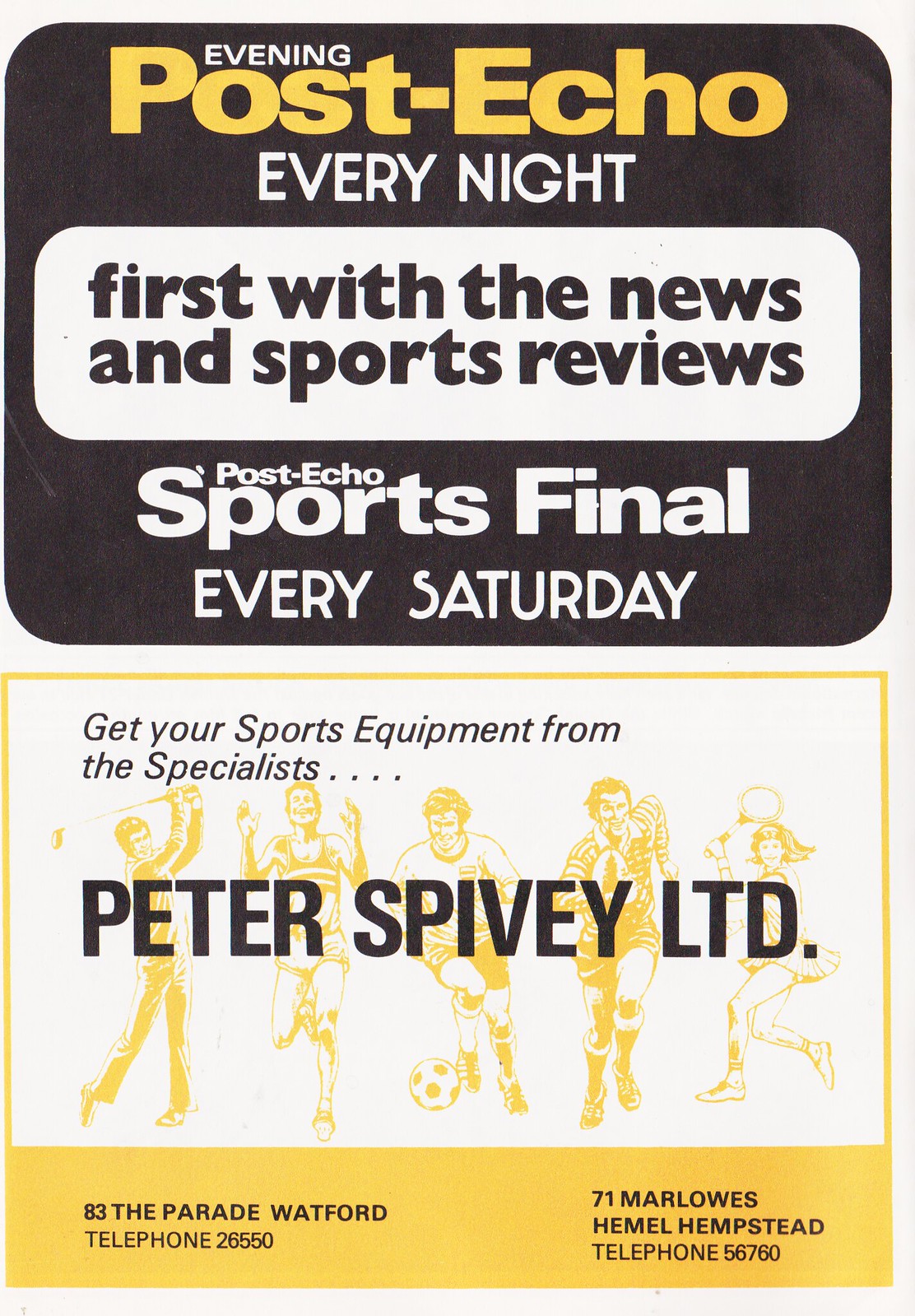This image features a detailed advertisement for the Evening Post Echo, styled in a vintage aesthetic. The ad has a black background with a combination of white and yellow text. The top headline reads "Evening Post Echo Every Night," with "Post Echo" highlighted in yellow. Below this, a white text bubble states "First with the news and sports reviews,” and another section mentions "Post Echo Sports Finals Every Saturday."

Beneath this, there is a second advertisement for Peter Spivey LTD, specializing in sports equipment. This ad is bordered in yellow, with black text and features illustrations of five people engaged in different sports activities: a golfer, a track runner, a soccer player, another soccer player in motion, and a tennis player. The ad promotes getting sports equipment from "the specialist," Peter Spivey LTD, with locations listed as "83 The Parade Watford," and "71 Marlowe's Hemel Hempstead," including respective phone numbers. The composition and colors, predominantly black, white, yellow, and gray, emphasize the vintage and informational nature of the advertisement.